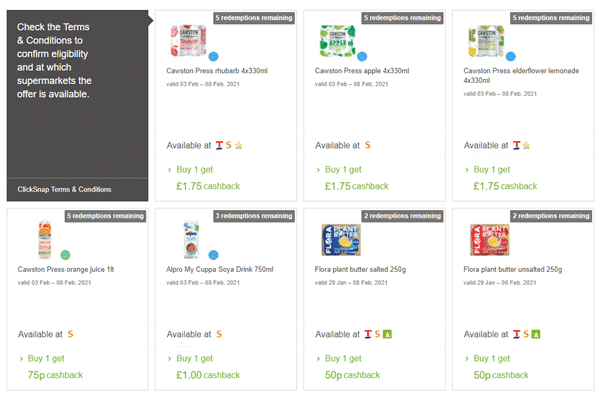Discover the terms and conditions to confirm your eligibility and find out which supermarkets offer this promotion. The items in question are as follows:

1. **Korshtun Purse Rubab** (4 cans, 330 ml each).
2. **Korshtun Purse Apple** (4 cans, 330 ml each).
3. **Korshtun Purse Elderflower Lemonade** (4 cans, 330 ml each).
4. **Korshtun Purse Orange Juice** (1 litre).
5. **Alpro Share Drinks** (750 ml).
6. **Flora Plant Butter Salted** (250 g).
7. **Flora Plant Butter Unsalted** (250 g).